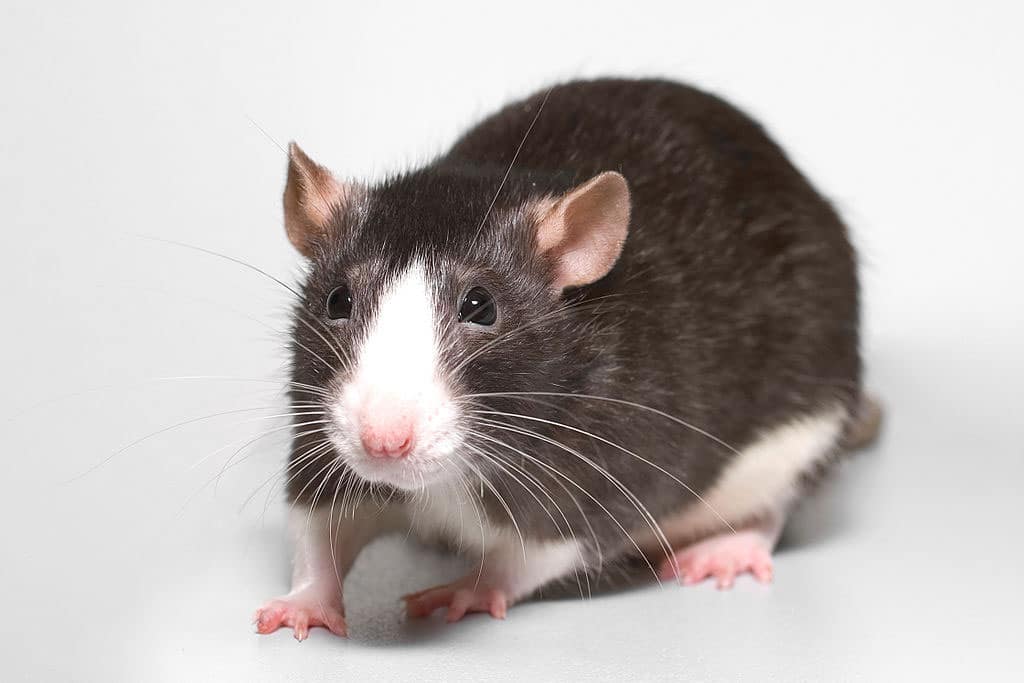This close-up photograph captures a pet rat facing the camera, giving a detailed and vivid view of its features. The rat sports a brown coat with a smooth, soft texture, contrasted by a white underbelly and white fur forming a distinct triangular patch that extends between its big, black beady eyes and down its muzzle. It has a pink, sensitive nose surrounded by numerous long, prominent whiskers sprouting in various directions. The rat's small, delicate ears are light brownish-pink, matching its petite pink feet. The image, reminiscent of a stock photo, is well-lit, casting a shadow behind the rat against a plain white cloth background, emphasizing the rat's pudgy, well-fed appearance. The rat appears slightly apprehensive, adding a touch of endearing charm to this highly detailed portrait.